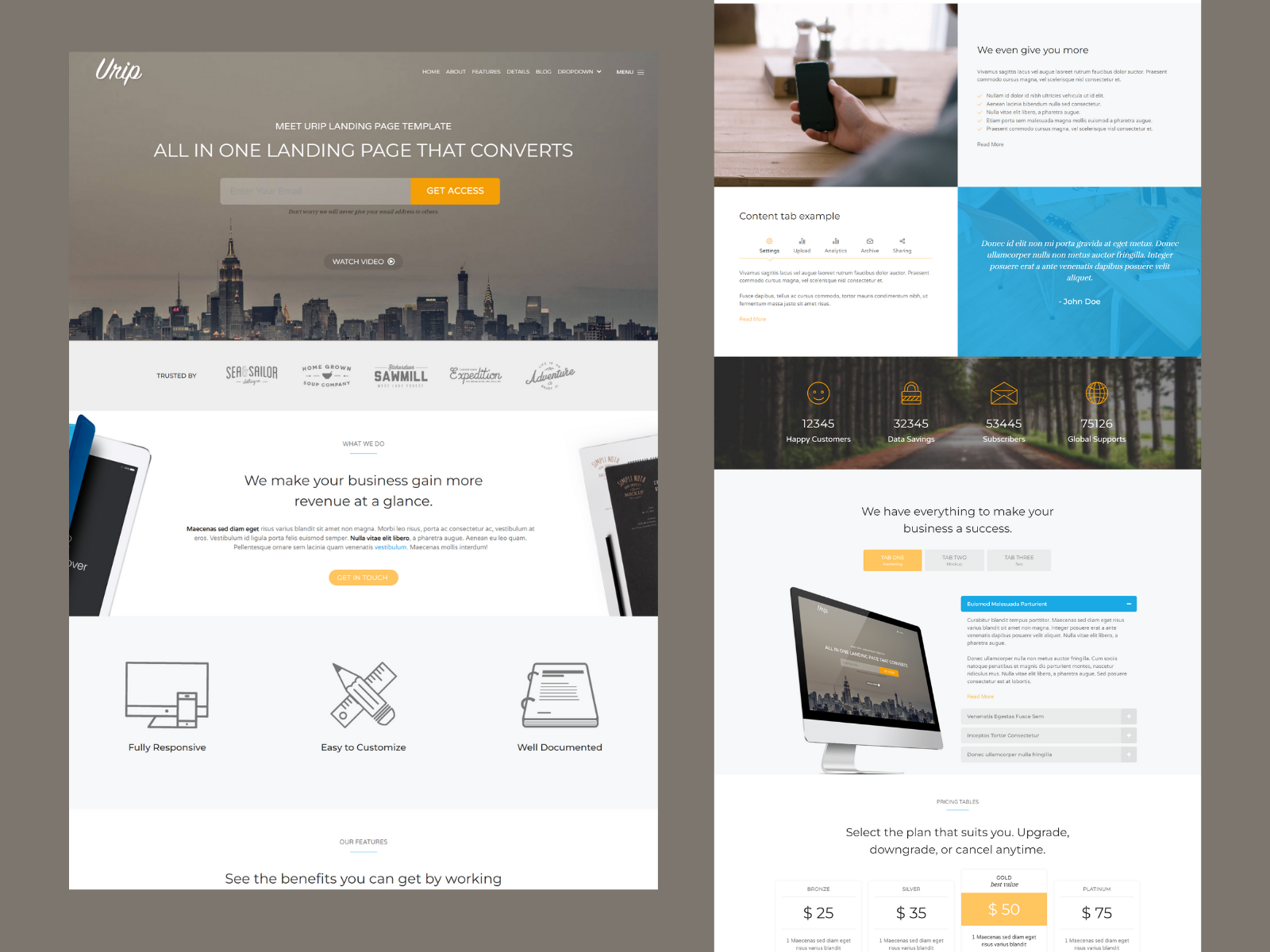**Detailed Caption:**

The image is a screenshot capturing various sections of a website. On the left side, at the top, it prominently displays the heading "All-in-One Landing Page That Converts." Below this heading, there's a central text box presumably containing persuasive content or a value proposition. Directly beneath this text box sits an eye-catching orange button labeled "Get Access." 

Below this section, another highlighted area reads "We Make Your Business Gain More Revenue at a Glance." This portion provides a quick overview, featuring several tabs with labels such as "See," "Think," "Web Documented," "Easy to Customize," and "Fully Responsive," which likely describe the website's features or services.

The right side of the screenshot shows a different part of the website, with much smaller text giving a more thorough description of the business. This section aims to provide detailed information about the company and its offerings.